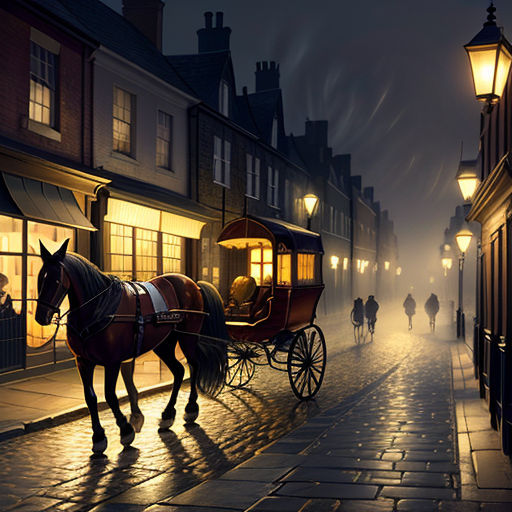The image is an AI-generated artistic illustration depicting a historical European street scene, likely set in the 1800s or earlier. The cobblestone road is wet and glistening under the night sky. On the left side of the foreground, there is a horse-drawn carriage, although there is nobody in the carriage or directing the horse. Interestingly, the horse appears to have five legs. The scene is illuminated by several street lamps, casting a blue, gold, and gray palette that contributes to the foggy, dreary atmosphere. Smoke billows from the chimneys of several buildings lining both sides of the street, with the lights on in most of them, suggesting life inside. The buildings are numerous and stretch as far as the eye can see, hinting at the expanse of the town. The street is devoid of people, adding to the somber and mysterious mood of the scene.